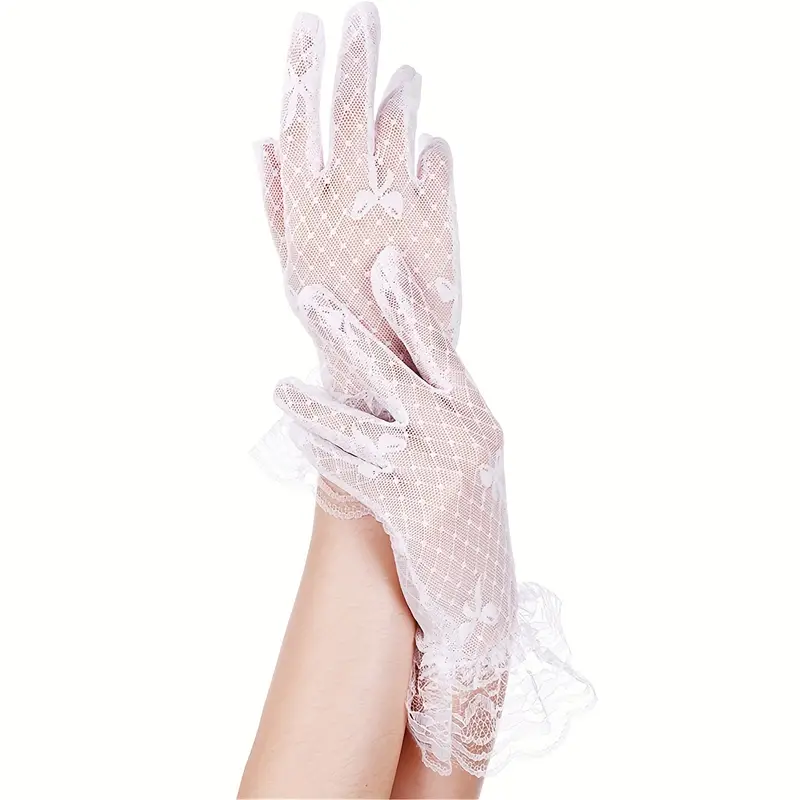In this close-up photograph, we see a pair of delicate, fair-skinned hands clad in intricate, white, lace gloves. The back of both hands is visible against a seamless white background, possibly photoshopped for a cleaner look. One hand is elevated, while the other grasps its wrist. The gloves are sheer, allowing the skin tone beneath to subtly show through, and feature an elaborate crisscross pattern reminiscent of bridal gloves. The end of the glove on the wrist is adorned with more pronounced, lacy fabric that flares out slightly, and is decorated with small, white ribbons or bows. Additionally, the gloves' detailed designs are concentrated particularly around the fingertips and areas showing wear. The composition focuses solely on the hands and a small section of the forearms, emphasizing the elegance and intricacy of the lace gloves amidst the stark, white backdrop.